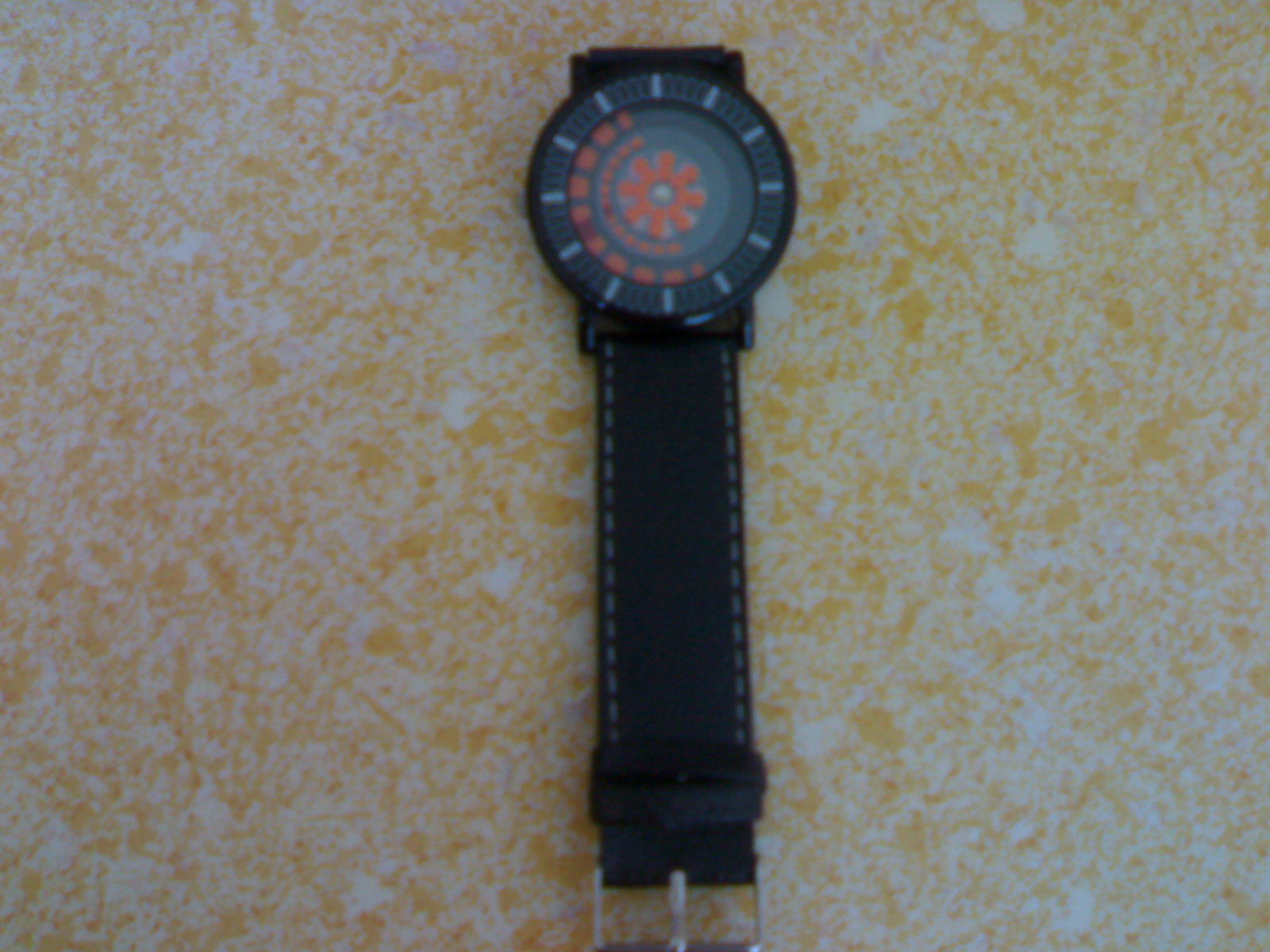This is a slightly blurry photograph of a wristwatch resting on a speckled counter that features yellow and white patterns. The watch boasts a black band with meticulously detailed gray stitching on both edges, and it is secured with a sleek silver latch. One side of the band is thoughtfully tucked underneath the watch itself. The watch face eschews traditional numbers in favor of minimalist tick marks. Its centerpiece is an intricate flower-like design, emanating a vibrant orange hue around a soft light gray core. Surrounding this central motif is a semicircle of smaller orange tick marks, which are, in turn, framed by a larger semicircle of more prominent orange tick marks. Completing the design is the watch's outer rim, finished in black with subtle gray tick marks.